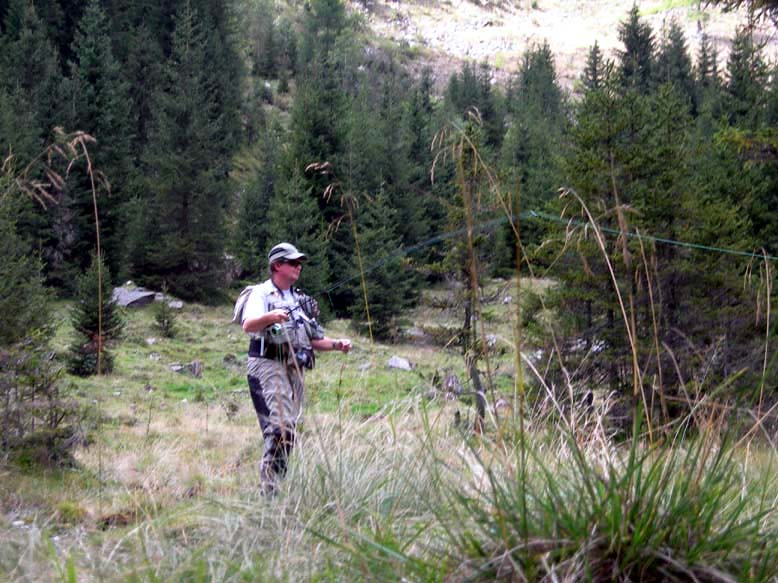In this detailed outdoor scene, a man stands centered in a predominantly flat, grassy field with a slight incline. The field, dotted with overgrown areas especially in the right-hand corner, stretches towards a dense forest of pine trees, some with green pine needles towering in the background. The entire setting is alive with natural elements, including rocks and boulders scattered across the terrain, all set against what appears to be the base of a mountain slope. The man, dressed in camouflage with a gray hat, sunglasses, and a backpack or vest over a white t-shirt, wears tan pants and is engrossed in an activity that seems to involve a long rod and an extended fishing line, indicating he is likely fly fishing. Despite the absence of visible water, the well-extended fishing line hints at a hidden stream or pond nearby, capturing the essence of a peaceful midday hunting or fishing escapade in the wilderness.